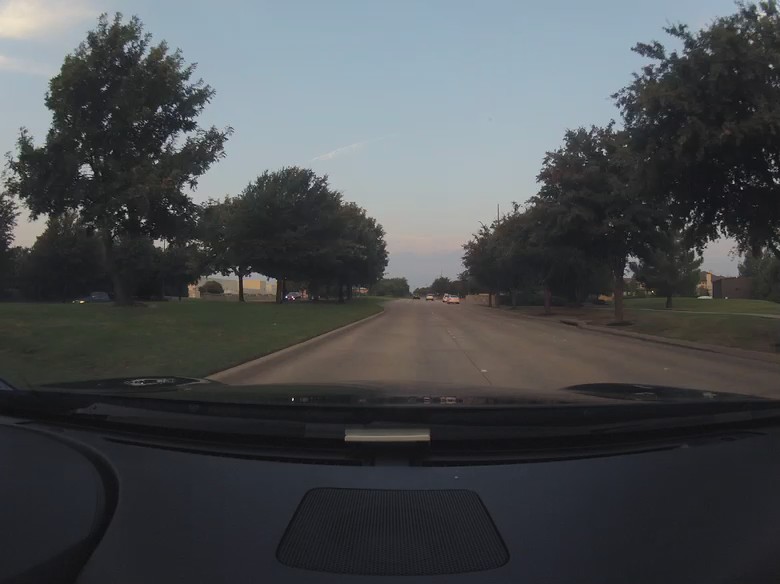Captured from the driver's seat inside a car, this image showcases a straightforward city road through the windshield, with the dashboard and windshield wipers framing the scene. The paved road extends straight into the distance, flanked by two flat areas on either side. Although typical for a city road, it notably lacks any dividing lines. The left and right sides of the road are lined with trees, which are positioned closer to the center rather than by the curbs. In the distance, a few cars and buildings punctuate the stretch of asphalt, adding depth to the urban landscape.